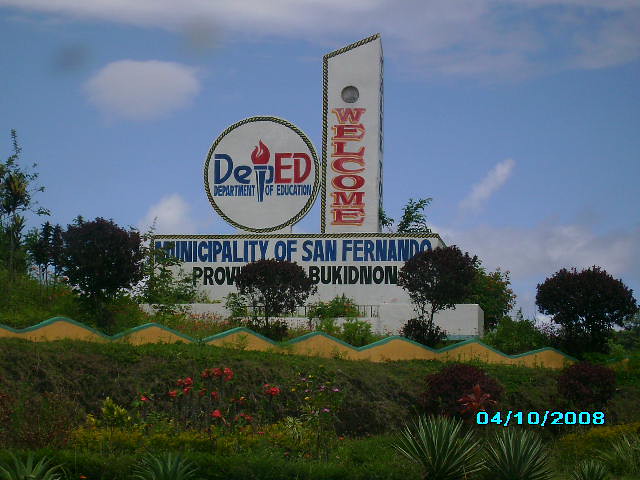The image captures a carefully manicured hillside adorned with vibrant flowers, bushes, and a small jagged yellow and green fence. Dominating the scene is a large rectangular monument that begins at the ground and stretches horizontally, its prominent blue text reading "Municipality of San Fernando" and black text indicating "Province of Bukidnon." Above it, a white circular sign with blue and red text announces the "Department of Education" with a central torch emblem. To the left side, a vertical obelisk features the word "Welcome" in bold red text on a white background. All these elements are set against a backdrop of a clear blue sky with scattered clouds. The image is date-stamped in mint green at the bottom right corner, indicating "04/10/2008."